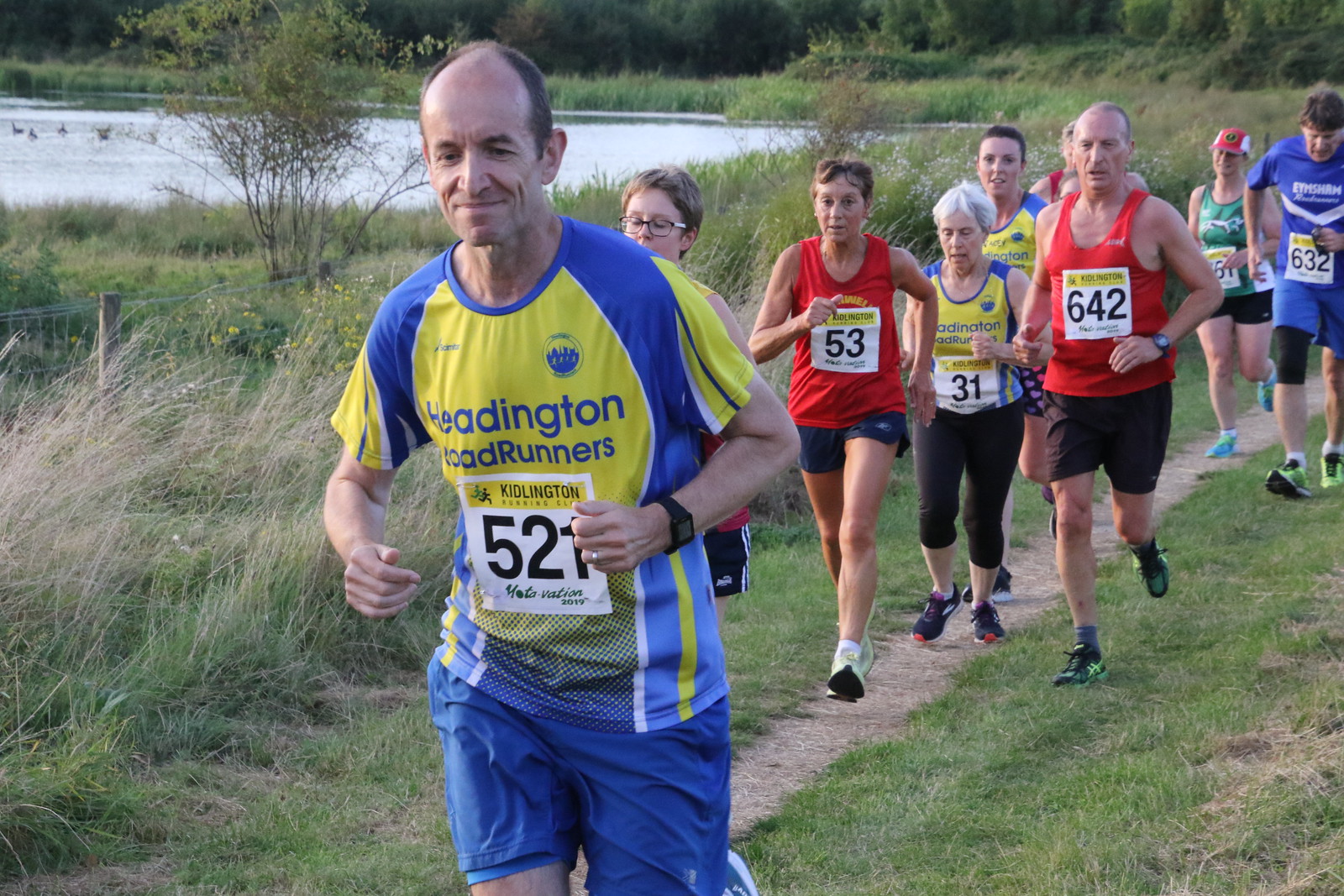In the image, a diverse group of around ten people jogs on a narrow dirt country path, their feet kicking up dust and dirt. Leading the pack is an older, balding man, distinguished by his yellow and blue jersey that reads "Reddington Roadrunners" and the number "521" on a white race bib attached to his shirt. He pairs this with blue shorts. Behind him, partially visible, is a woman with short hair and glasses, followed by other runners clad in a mix of red, blue, green, and additional yellow and blue outfits. They jog through a verdant, grassy landscape that meanders around a reflective body of water in the far background, appearing light blue and whitish under the sunlight. Beyond the water, a dense tree line with lush green foliage outlines the horizon, framing the scene in natural beauty. The overall ambiance suggests the runners are participating in a marathon or race amidst the serene, picturesque setting of a wooded countryside.